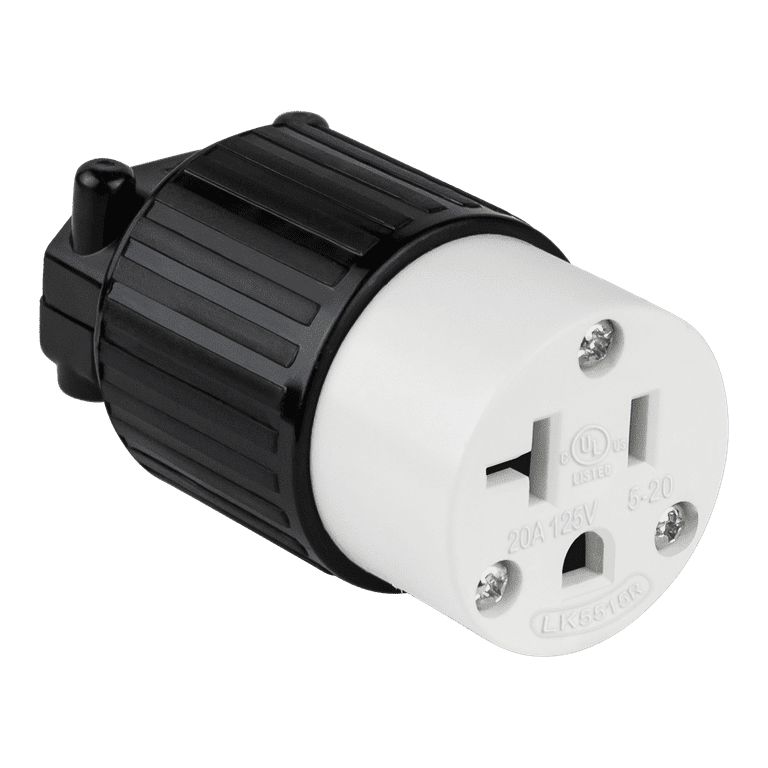The photograph features a close-up view of an electrical outlet converter, set against an all-white background, making it appear like a stock image typically used on a product page. The converter has a cylindrical design with distinct sections. The front part of the converter is white and houses three holes configured to accommodate a three-pronged plug. One of the holes has a slit extending towards the left. You can see three silver screws on the front—one at the top and two in the bottom corners—securing the device.

Prominently displayed on the white front are multiple inscriptions. Near the center, there's a circle with the letters "UL" inside, followed by the word "Listed" underneath it. Further below, in larger text, it reads "20 Amp, 125 Volt, 5-20." At the very bottom, the serial number "LK5515R" is printed.

The base of the converter, distinctively black, features textured lines designed for an easy grip when unplugging. Behind the black textured section, there's an additional smaller black section, cylindrical in shape, possibly indicating where it connects to a wall or another device. The combination of white and black sections makes the converter functional and visually identifiable.